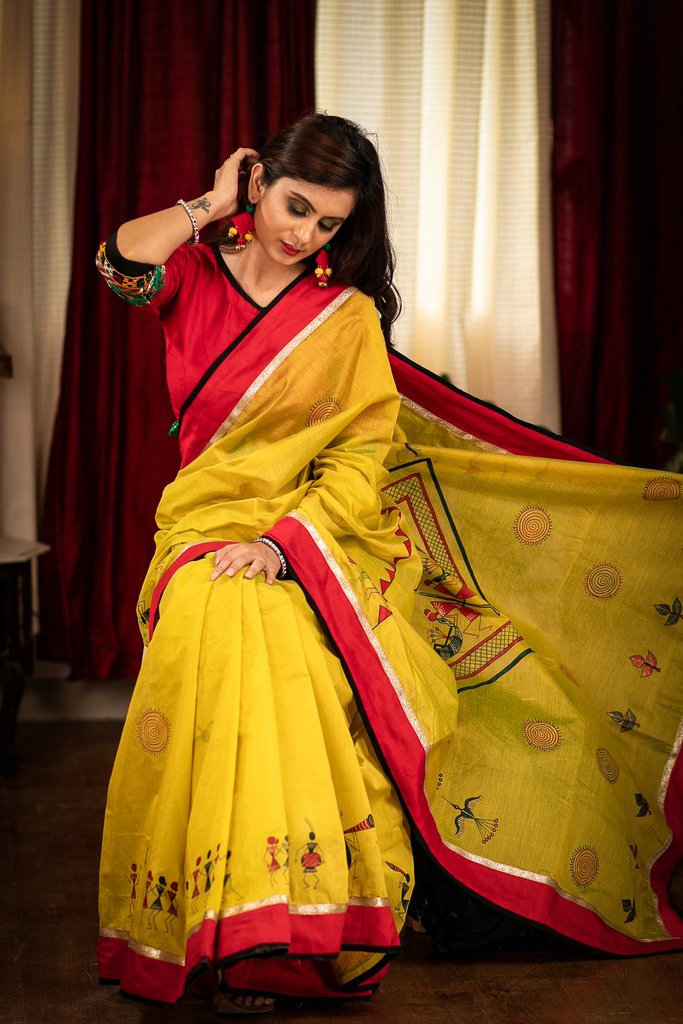This is a photograph of a very beautiful Indian woman sitting on the arm of a sofa in a room with rich decor. She has long, shiny, wavy dark brown hair and dramatic makeup with smoky gray eyeshadow and bright red lipstick. Her eyes are closed, and her head is slightly tilted to her left as she demurely looks down at the ground. Her right arm is gracefully bent, tucking her hair behind her ear, revealing a subtle wrist tattoo and two bracelets—one appearing to be pearl, the other a diamond bangle. Her left hand rests gently on her knee.

She is adorned in a traditional sari, an exquisite piece of attire that features a lengthy, flowing fabric draped around her. The primary color of the sari is a mustard yellow with intricate patterns, including representations of birds, people dancing or playing instruments, leaves, suns with spiraling centers, and other cultural symbols. The sari has a V-neck with a distinctive black, red, and white trim. The upper portion of the dress is predominantly red, complementing the yellow and white borders that run throughout. There is a cape-like section extending to her left, presenting more detailed patterns. Her sari is also embellished with a red border and gold trim.

She accessorizes with bold, long dangling earrings that feature red diamond shapes with yellow circles at the bottom. Behind her, a large window is framed by wide vertical stripes of deep burgundy red and white curtains, creating a rich backdrop. The floor underneath is a dark red or maroon carpet, contributing to the overall luxurious and warm ambiance of the scene.